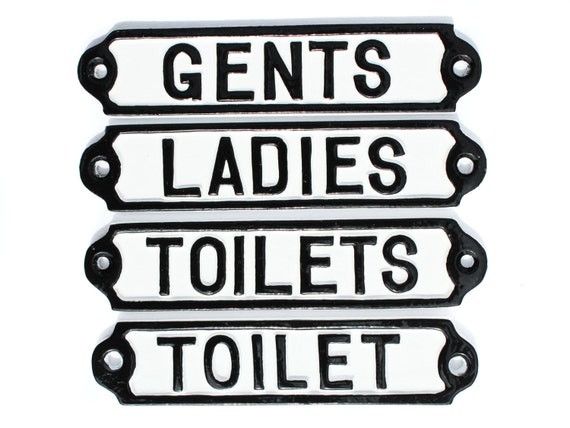The image displays four horizontally-aligned, rectangular metal signs with rounded sides, each bordered in black with a central white background. Each sign is equipped with screw holes on either end for mounting purposes. The signs are designated for a public establishment, likely a restaurant or similar venue, indicating restroom facilities. The top sign reads "GENTS," followed by "LADIES," then "TOILETS," and the bottom one "TOILET," all in capital black raised lettering. The image is oriented in portrait mode, showcasing the signs stacked one above the other, ready for installation.